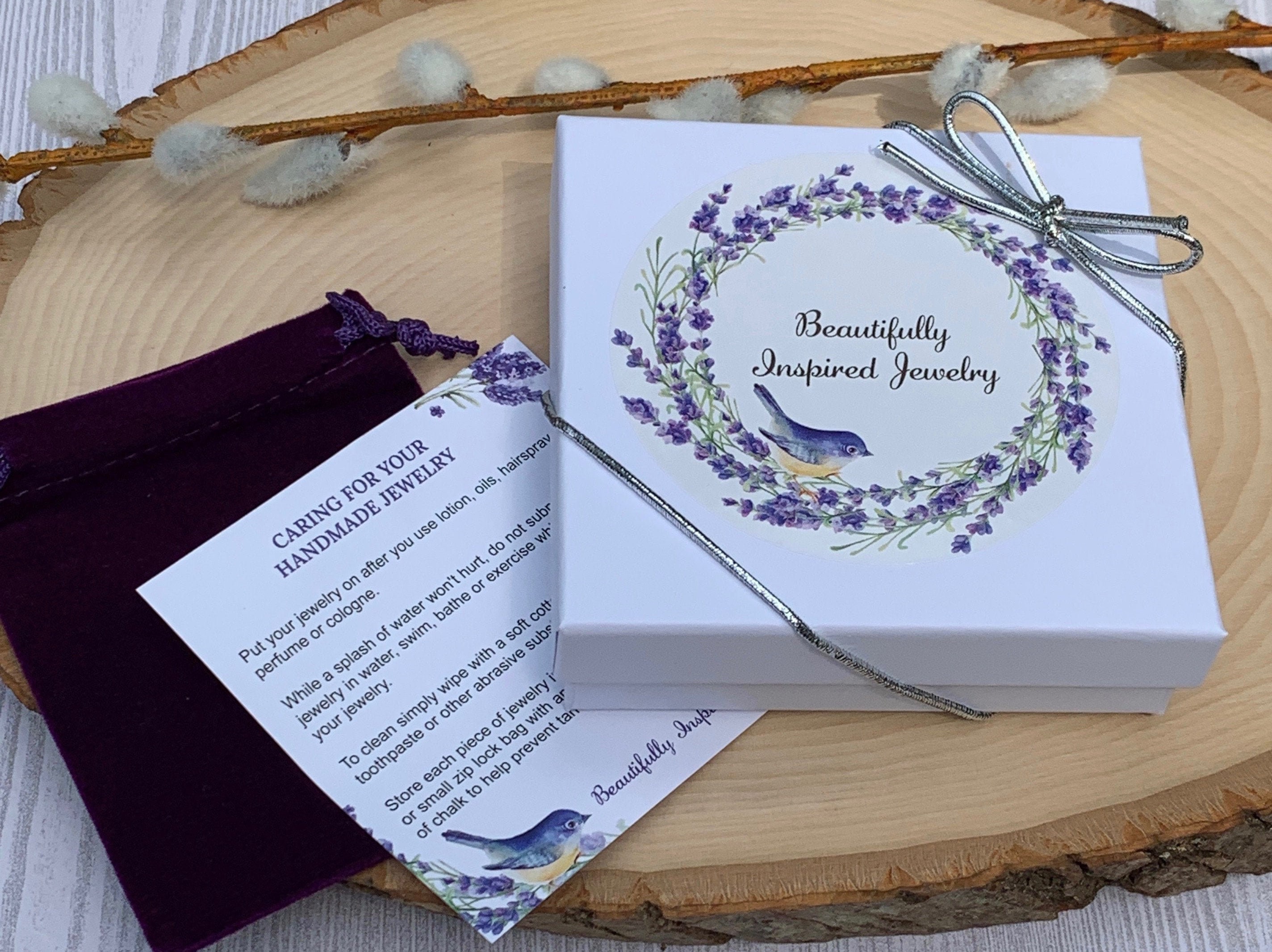The image is a meticulously arranged promotional photograph for a jewelry product, likely intended for use in an online shop listing or catalog. Central to the image is a white flat box with a lid secured by a silver drawstring, and adorned with a white sticker that features the text "Beautifully Inspired Jewelry." Surrounding this text is a delicate wreath of purple flowers, with a small bird perched on it, contributing to a charming, rustic aesthetic.

The box rests atop a circular wooden slab, showcasing the natural grain and bark of the wood, which sits on a table with a whitewashed, vertical pattern. A stalk of a plant resembling cotton, or possibly pussy willows, is artfully placed across the top of the slab to add a touch of organic elegance to the scene.

Partially tucked under the box is a white piece of paper that provides detailed care instructions for the handmade jewelry. The paper mirrors the box's decorative theme, featuring similar purple flowers and the same little bird in the corners. Alongside, a velvet pouch is subtly visible, suggesting it is intended to house the jewelry.

Together, these elements create a cohesive and inviting display, emphasizing the product's artisanal quality and the careful attention to detail in both the packaging and the presentation.